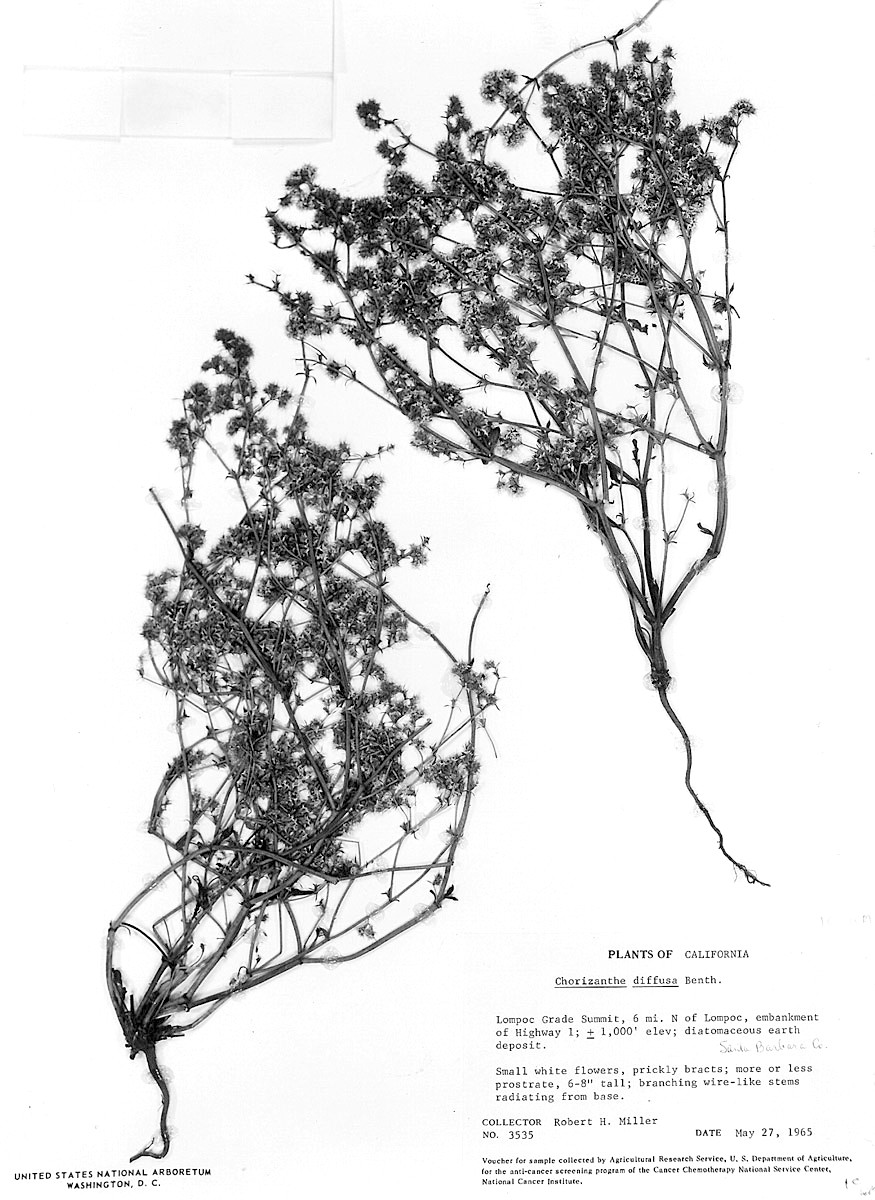This black and white image depicts two botanical specimens presented against a white background, giving the impression that they were taken from a book or catalog. Each plant starts with a thin root system at the base, from which multiple slender branches extend. These branches bear numerous tiny structures that could be leaves or flowers, difficult to discern due to the monochromatic nature of the photo. 

The specimen on the right rises from the bottom to the top of the image, while the second one is located in the lower left corner. Below the left specimen, text reads "United States National Arboretum, Washington D.C." To the lower right of the image, the text states "Plants of California," followed by the plant's scientific name, "Corazanth diffusa Benth." Additional information includes the collector's name, "Robert H. Miller," the identification number "3535," and the collection date "May 27, 1965." The image also features some smaller printed text describing the plant's characteristics and other botanical details.